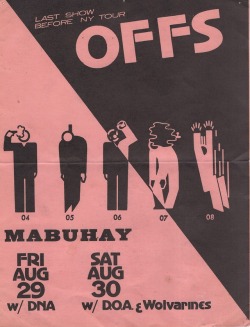This advertisement poster for a concert or performance features a striking design split diagonally into black and a light peach-pink colors. Dominated by dramatic visuals and text, the poster announces, "Last show before NY tour," highlighting the band name "OFFS" in bold, capital letters. The central part of the poster displays five stylized human figures, each marked with the numbers 04, 05, 06, 07, and 08. Figure 04 appears to be shooting itself in the head, while figure 05 seems to be hanging by the neck. Figure 06, divided into black and white halves, lifts a cup, making it unclear whether it's drinking. Figure 07 is bent over, touching one knee, with a dark cloud hovering above its head. Figure 08 looks to be falling with motion lines accentuating the descent, arms outstretched, and fingers splayed. At the bottom, it says "Mabuhay," a Tagalog greeting meaning "live" or "hello." The dates and supporting acts are noted: Friday, August 29th with DNA, and Saturday, August 30th with DOA and the Wolverines.